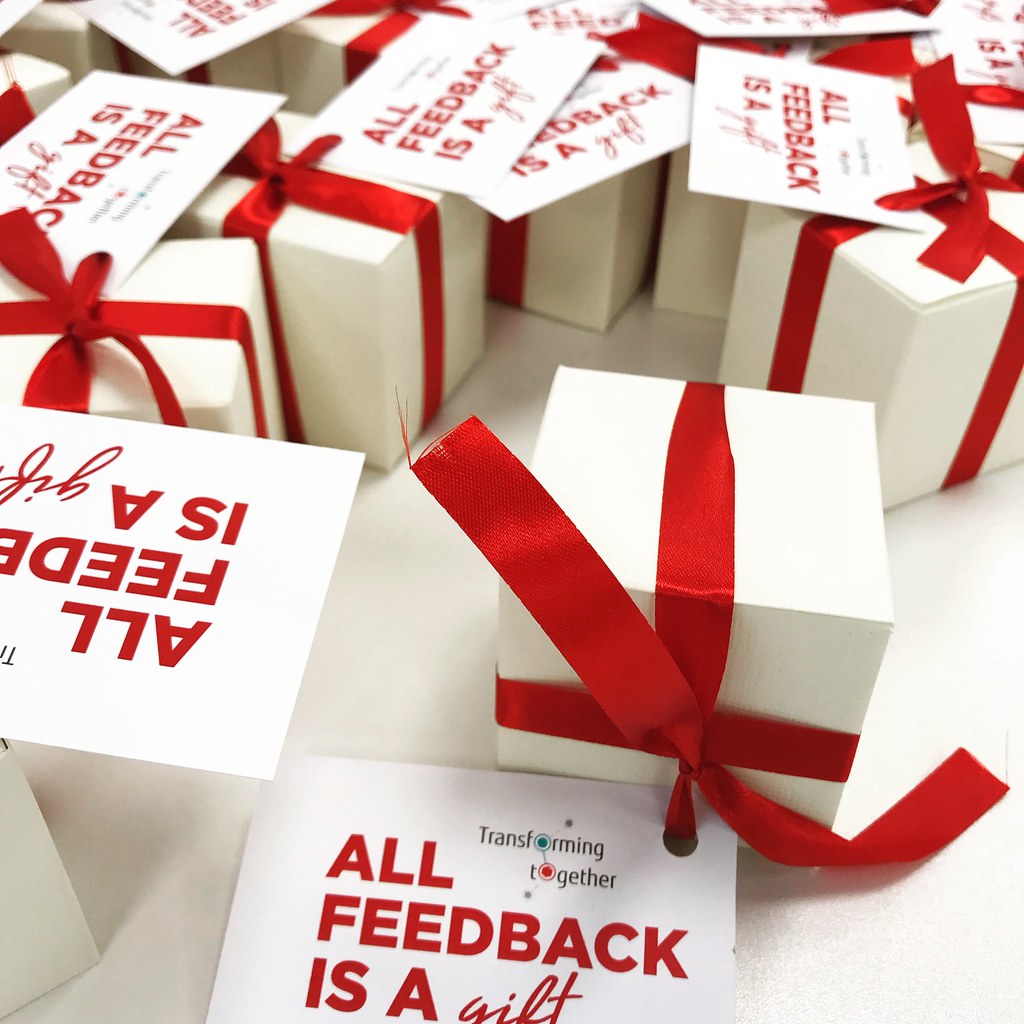The image depicts approximately 10 to 12 perfectly square white boxes, each measuring around six by six inches. All the boxes are uniformly adorned with red ribbons that wrap around each side, creating a cross pattern on the top where the ribbons are tied. Attached to each ribbon is a white tag with bold red lettering that reads, "Transforming together. All feedback is a gift." Notably, the 'O' in "transforming" is green, while the 'O' in "together" is red, adding subtle color variations to the text. The boxes are scattered across a white surface, with some toppled over and others standing upright, presenting a random but visually engaging arrangement.